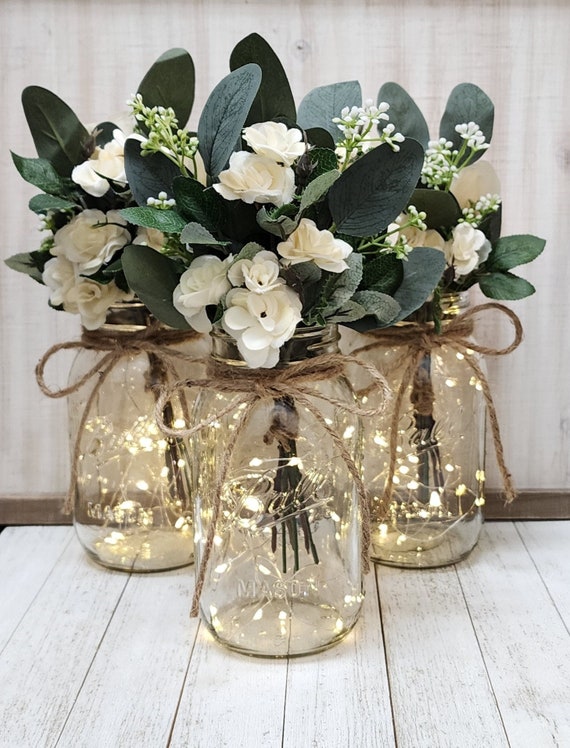The image is a highly detailed color photograph in portrait orientation, showcasing a trio of elegant glass Ball Mason jars arranged in a triangular pattern on a wooden surface with vertical white planks. The central jar is positioned closest to the viewer, with two jars flanking it slightly behind on either side. Each jar contains a carefully arranged bouquet featuring clusters of small white flowers, baby's breath, and dark green leaves, giving the appearance of well-coordinated floral displays, though it's unclear whether the plants are real or artificial. Illuminating the scene, delicate white Christmas lights are nestled inside each jar, casting a soft, bright glow that enhances the overall aesthetic. The lights are tiny and elegant, strung together on a wire, emphasizing their intricate detail. Complementing the rustic charm, each jar is adorned with a piece of beige twine tied into a neat bow around the neck, its free ends hanging gracefully. The iconic "Ball" logo is raised and italicized on the front of each jar, contributing to the classic, homely feel of the composition.